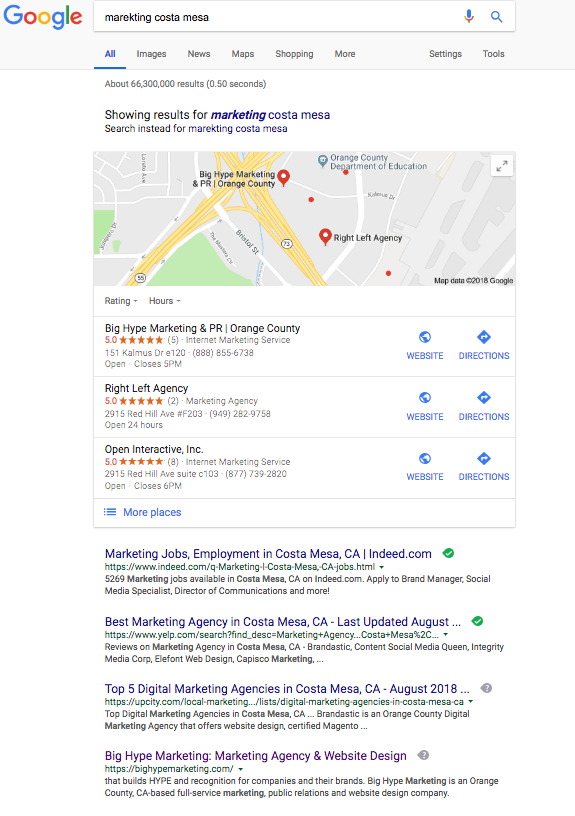This is a detailed, cropped image of a Google web search interface from a desktop computer. Located in the top left corner is the recognizable Google icon, with a search bar positioned to its right displaying the query, "marketing costa mesa" in lowercase letters. Beneath the search bar, a line of text reads, "Showing results for marketing costa mesa, Search instead for marketing costa mesa," redundantly.

Below this text, a prominent map occupies a significant portion of the screen, dotted with red pin drops indicating various business locations around Costa Mesa. Following the map is a vertical listing of search results. The top three results correspond to the pins on the map and include detailed information: the name of each business, star ratings denoting their quality, their physical addresses, and their hours of operation. To the right of each business listing are icons for a website and directions, both hyperlinked in blue for easy access.

At the bottom of the map section, to the left, there's a clickable link labeled "More places," providing the option to expand the list. Just beneath this, the page displays four text entries, all highlighted in blue, functioning as additional links. Among these entries, the top two feature a green checkmark on the far right, signifying that these businesses are verified.

This cleaned-up description offers a comprehensive view of the cropped Google search image while maintaining a high level of detail.